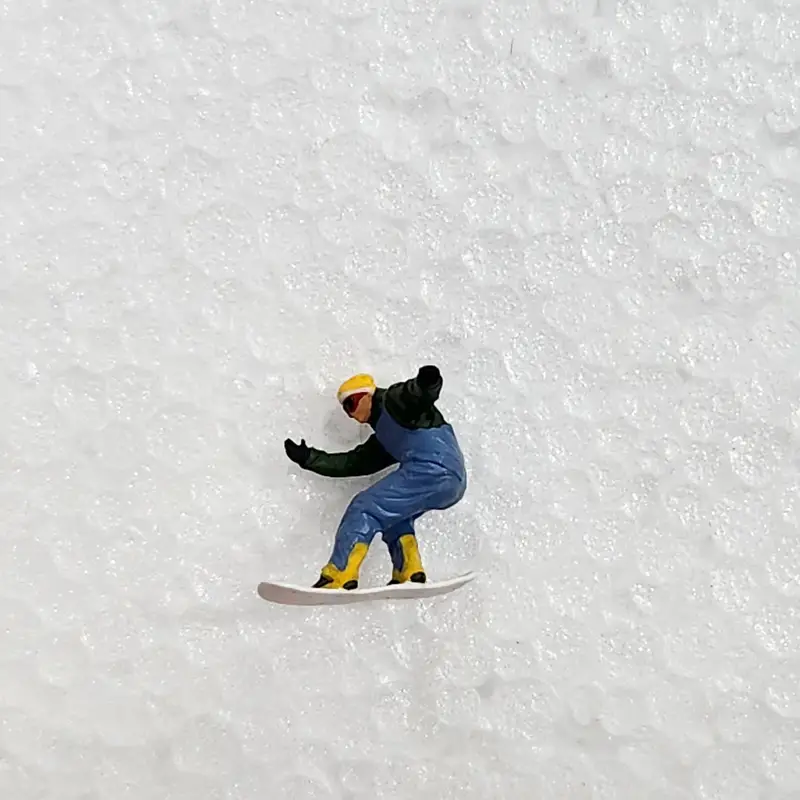In this colored photograph, a detailed handmade clay figurine of a man snowboarding is prominently displayed against a textured white background that resembles ice and snow. The figurine features striking attire: a blue pants and blue vest over a black jacket, completed with black gloves. He sports black and yellow snow boots, red and black goggles, and a yellow and white ski cap. His skin tone is light. The figurine appears in motion, with arms outstretched as if gliding from right to left across the image. The snowboard beneath his feet is distinctly white, and the background is notably flat with small round patterns, enhancing the icy, shiny effect. The craftsmanship of the figurine, combined with the realistic portrayal of snow and motion, gives the image a dynamic and lifelike quality.